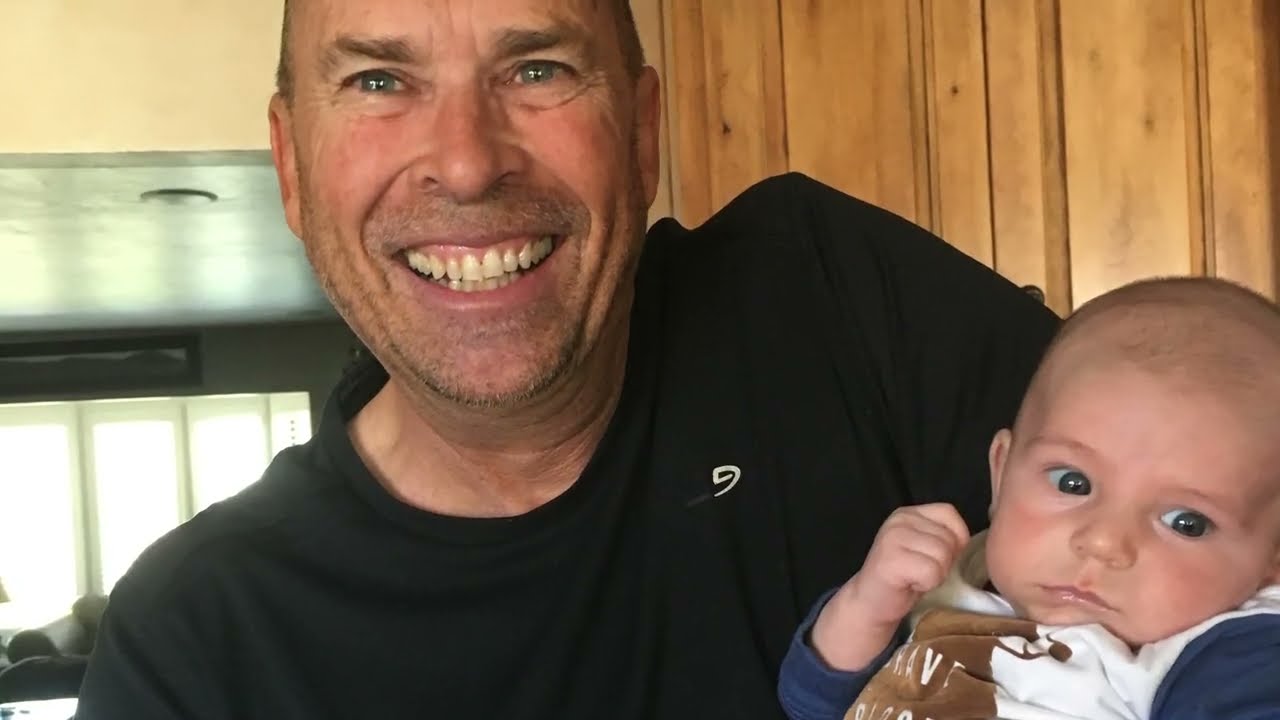In the photograph, an older Caucasian man, likely in his late 50s or 60s, is proudly holding a baby. The man's head is slightly cropped by the camera, revealing short and thin hair on the sides. With a bright, large smile that exposes both his gums and lower teeth, his happiness is evident. He has blue eyes and wears a black crewneck shirt. His left shoulder is raised as if he is presenting the baby to the camera.

The baby, also Caucasian, has blue-gray eyes and a mostly bald head. He is dressed in a blue shirt with a white and brown bib. Positioned in the lower right corner of the image, the baby seems to be looking toward the lower right, appearing not entirely happy. The background features wooden paneling, a window with black framing, and sunlight filtering through, providing a warm ambiance to the scene. The image captures a heartwarming moment between the man, possibly the baby's proud father or grandfather, against a homely backdrop.